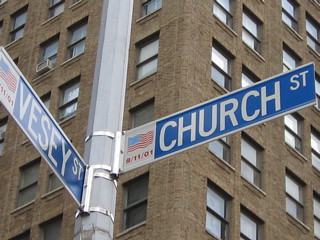This color photograph captures the intersection of Church Street and Vesey Street, marked by distinctive street signs mounted on a tall, thick pole toward the center left of the image. The background is dominated by a tall building with brown brick walls that catch the eye due to their textured façade. The building features numerous small, squarish windows, each divided into two panes, creating a grid-like pattern across the structure. We seem to be viewing this scene from a vantage point that highlights the corner of the building. The street signs themselves are notable for their detailed design: each has a white edge adorned with an emblem resembling a US flag in blue and red, along with some red text beneath that is not entirely legible. The main body of the signs is blue with prominent white lettering, clearly identifying Church Street on the right and Vesey Street on the left. The windows in the immediate background underneath the street signs appear darker, in contrast to others that reflect light, adding a dynamic quality to the composition.